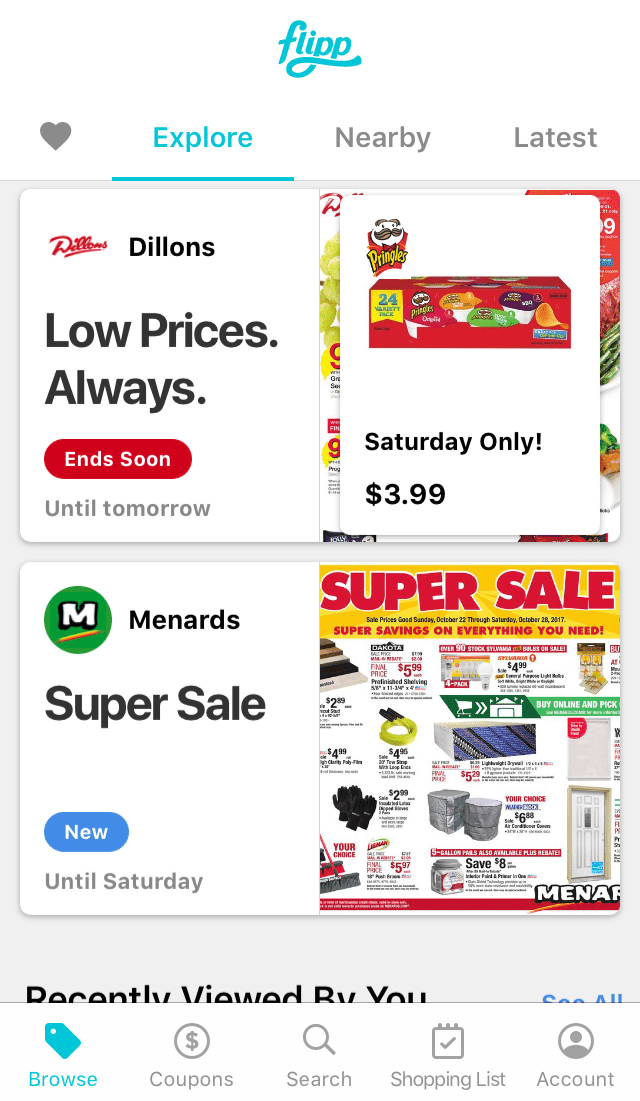This image appears to be a screenshot of a website aimed at helping users find cheaper products through various sales promotions. The top of the page features a blue, cursive logo reading "FLIPP". A navigation bar with icons and options such as a heart icon for favorites, and links labeled "EXPLORE," "NEARBY," and "LATEST" follows the logo.

Beneath the navigation bar, the page displays four promotional images arranged in a 2x2 grid. The top-left image showcases a deal labeled "DYLAN'S LOW PRICE AS ALWAYS" with an accompanying red button indicating "IN SOON" and a note that the offer lasts "UNTIL TOMORROW." 

On the top-right, there is another promotion labeled "SATURDAY ONLY." Below, the bottom-left image advertises the "MENARD SUPERSALE" with a note that it is "NEW UNTIL SATURDAY." The bottom-right image features a label "SUPERSALE" along with various displayed products, and a note indicating they were "RECENTLY VIEWED BY YOU."

At the bottom of the page, there is another menu with options labeled "BROWSE," "COUPON," "SEARCH," "SHOPPING LIST," and "ACCOUNT," enabling users to navigate and utilize the various features of the site.